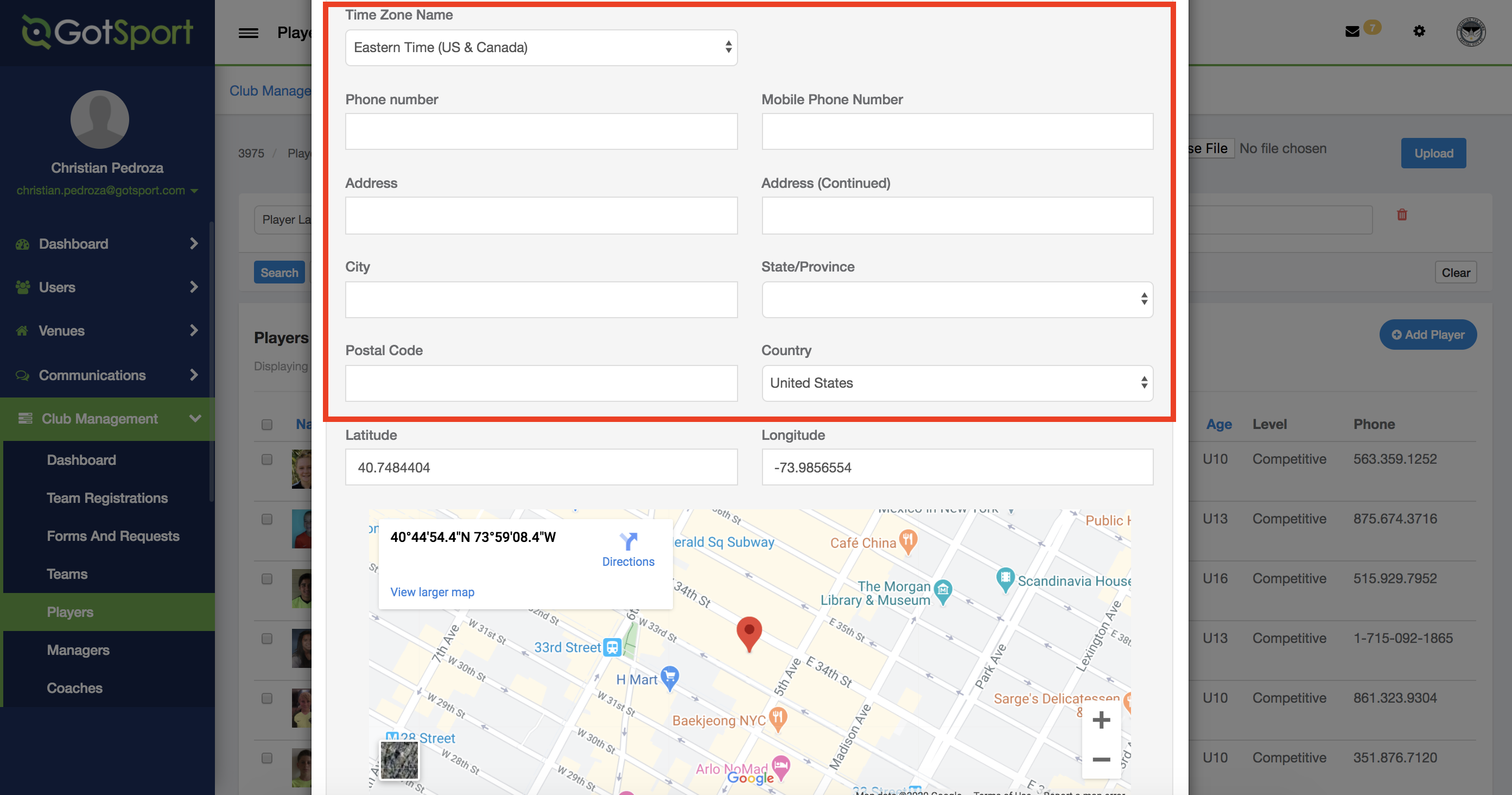In the image, the left-hand column prominently displays the word "Godsport" with "God" in white text and "sport" in green text. To the left of the word is a distinctive logo consisting of two circles: the upper part is tilted with a line forming a semi-circle, and the lower part is a lighter green circle with a dot in its center.

Below this, the username "Christian Pedroza" (spelled P-E-D-R-O-Z-A) is shown, indicating the user is logged in. The user's email appears to have a connection to GetSport, as inferred from the latter part of the email. 

The interface features a dashboard with expandable options including "User," "Venue," and "Communications." The "Club Management" section is currently highlighted in green. Within the "Club Management" section, there are various categories listed: Dashboard, Team Registrations, Forums, Requests, Teams, Players, Managers, and Coaches, with the present focus being on "Players."

A dialog box has appeared overlaying the information in the background, titled "Time Zone," set to Eastern Time Zone (U.S. and Canada). The box contains fields for entering details such as phone number, address, city, postal code, mobile phone number, state/province (accessible via a dropdown menu), and country. Additionally, it features input fields for latitude and longitude, alongside a Google Maps display showing various locations within the city.

Behind the dialog box, partially visible, are thumbnail pictures and details of several players, including their ages and phone numbers, suggesting a section focused on kids participating at competitive levels. The thumbnails are displayed in a column labeled with names.